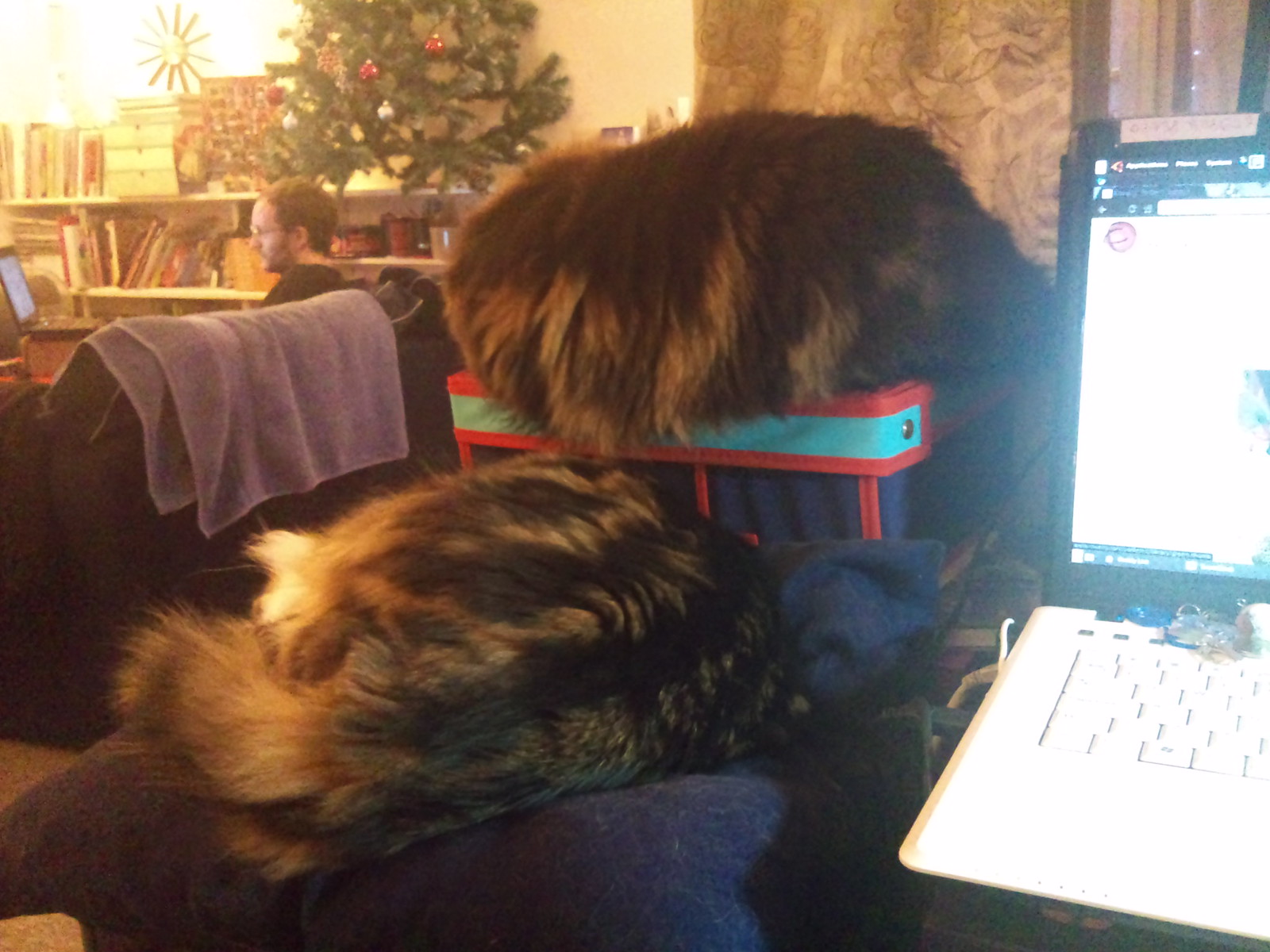The photograph captures an indoor cafe setting characterized by cozy and eclectic elements. Central to the image is a plush blue chair that serves as a lounging spot for two large, long-haired tabby cats, possibly Maine Coons. The cats, featuring a mix of dark brown, black, and grey fur, are curled up: one directly on the chair and the other atop a fabric box placed on the chair. Their faces are not visible, adding an enigmatic quality to their presence.

On the right side of the image, a bright laptop screen casts a glow over the keyboard and surrounding area, indicating it is in use. To the left, a black couch adorned with a purple towel on its backrest seats a Caucasian man engrossed in his own laptop. Behind him, bookshelves brimming with books stand out, crowned by a small fake Christmas tree that adds a touch of festive decor. The overall ambiance suggests a relaxed, communal hangout spot, though the spaciousness makes it clear it's likely a cafe rather than a private living room.